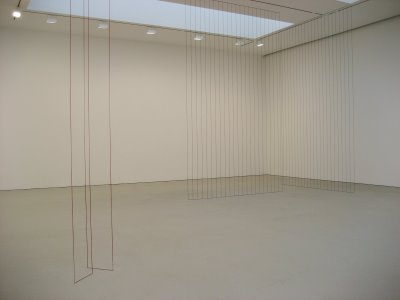The image depicts a minimalist, modern abstract art installation set in an almost empty room with stark white walls and a light gray concrete floor. From the ceiling, numerous thin strings or wires hang, almost reaching the floor. On the left side, four wires are visible, with two forming a rectangle at the bottom. To the right, near the room's corner, two rectangular sheets formed by numerous vertical strings hang, creating a denser, curtain-like appearance. The ceiling at the back of the room features a large rectangular skylight or sunroof with a glowing blue hue, framed by seven small white recessed lights where the ceiling meets the wall. The stark, geometric elements and the play of light create a striking, almost ethereal atmosphere in the room.